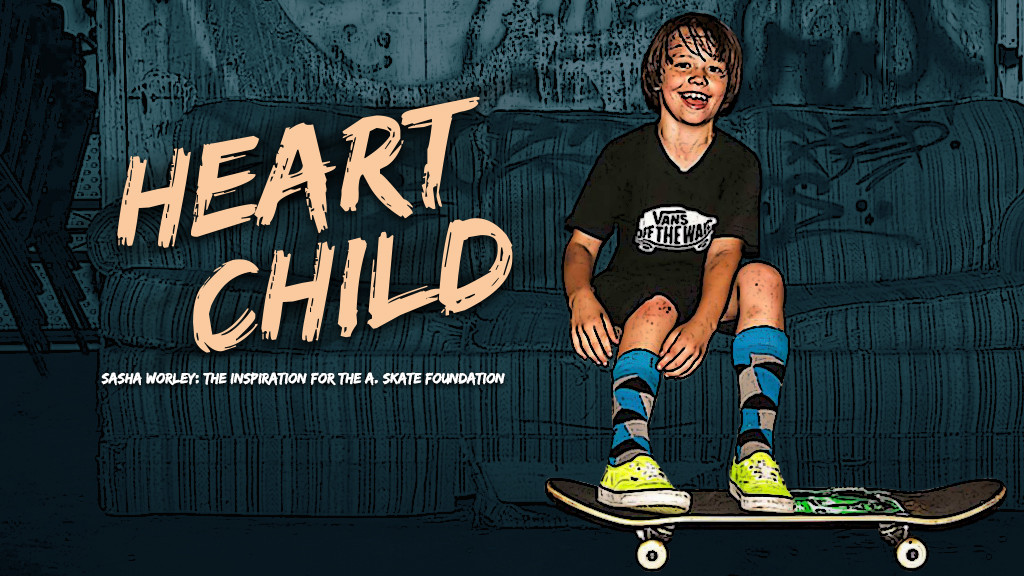The image is a color, photo-edited promotional photograph arranged in a horizontal, landscape orientation. The subject is a smiling, young Caucasian male, approximately 9-11 years old, with medium-length brown hair that falls around his face and tassel bangs over his forehead. He is seated on a blue-striped sofa, wearing a black Vans t-shirt with a white, somewhat indistinguishable logo on the chest, black shorts, blue long socks with a pattern, and light neon green sneakers. His feet rest on a skateboard, which is visible in profile at the bottom right of the image, featuring a dark gray deck with lime green edges matching his sneakers. The background of the image includes dark blue and black abstract designs, enhancing the graphic design elements. On the left side, in a beige handwritten-style font, are the words "HEART CHILD" arranged diagonally. Below these in white text, it says "Sasha Worley: The inspiration for the A. Skate Foundation."